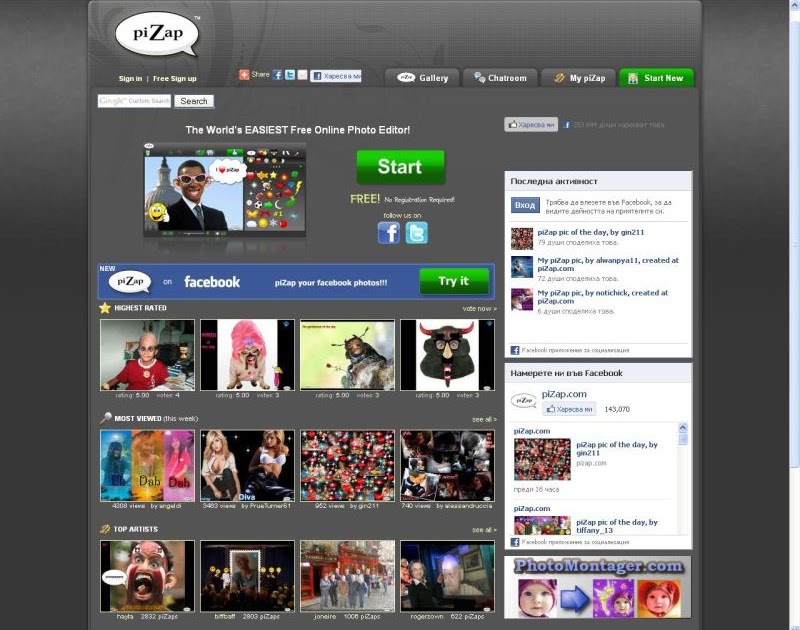This is a cropped screenshot of the PTZAP website. The visible portion of the screen excludes the very top of the browser and the bottom of the page, focusing mainly on the central area. The background of the webpage is black, creating a striking backdrop for the content presented.

At the top left of the screenshot, the PTZAP logo is prominently displayed within a comic-style speech bubble. Directly below this logo, small white text prompts users to "sign in," while nearby text states "free to sign up." To the right of these options, a series of icons for sharing and social media follow: a share icon, a Facebook icon, a Twitch icon, and a follow bar for Facebook.

The website navigation is housed on the right side, featuring four category tabs titled "Gallery," "Chat Room," "My PTZAP," and "Start New." 

Beneath this header section on the left, there is a search bar, facilitating easy navigation across the site. Centrally positioned below this header is a large advertisement claiming to be "the world's easiest free online photo editor," with an accompanying thumbnail. Further to the right of the ad, the words "Start" and "Free" draw the user's attention.

A prominent blue banner stretches across the screen just below the advertisement, encouraging visitors to "New PTZAP on Facebook. PTZAP your Facebook photos. Try it."

The screen's lower section showcases three rows, each containing four thumbnail images categorized under different headings. The first row is labeled "Highest Rated," the second row in the middle is titled "Most Views," and the bottom row is designated "Top Artists."